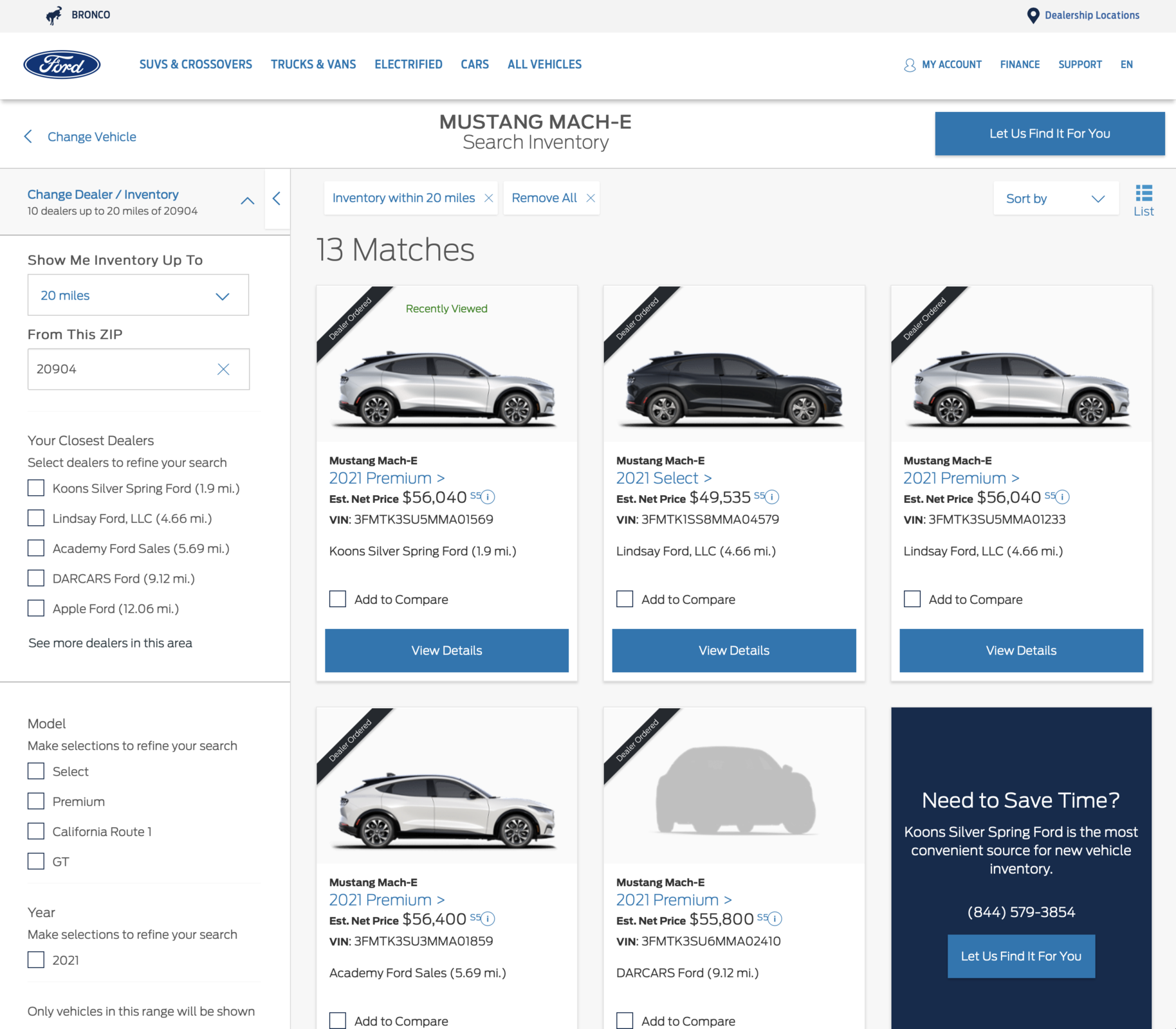Here is a detailed and cleaned-up descriptive caption for the provided content:

---

Screenshot of a Ford Motor Company Webpage

The screenshot features a webpage from the Ford Motor Company. At the top of the page is a light gray logo. On the left, the page displays the word "Bronco" alongside an icon of a horse. On the right, the text reads "Dealership Locations."

Below this header, a navigation bar stretches across the page. On the left side of the bar is the classic Ford logo. Next to it are several categories: "SUVs & Crossovers," "Trucks & Vans," "Electrified," "Cars," and "All Vehicles." On the right side of this bar, the options include "My Account," "Finance," "Support," and a language selection option marked "EN" for English.

Moving down, a prominent banner highlights the "Mustang Mach-E." In the center, it features an option to "Search Inventory." On the left side of the banner, there's a "Change Vehicle" option. On the right side, another option reads "Let Us Find It For You."

Below the banner, search results indicate that there are 13 matches. On the left-hand side, the filtering options include: "Show me inventory up to 20 miles from this zip code 20904." Listed below this are "Your Closest Dealers," followed by filtering choices for "Models" and "Years."

On the right side of these filters, there are five car listings followed by an advertisement. The first three listings on the top row display:

1. Mustang Mach-E 2021 Premium - Price: $56,040
2. Mustang Mach-E 2021 Select - Price: $49,535
3. Mustang Mach-E 2021 Premium - Price: $56,040

Below these, additional listings are:

4. Mustang Mach-E 2021 Premium - Price: $56,400
5. Mustang Mach-E 2021 Premium - Price: $55,800

Finally, an advertisement at the bottom promotes Kuhn Silver Spring Ford, stating: "Need to save time? Kuhn Silver Spring Ford is the most convenient source for your new inventory," and includes a phone number.